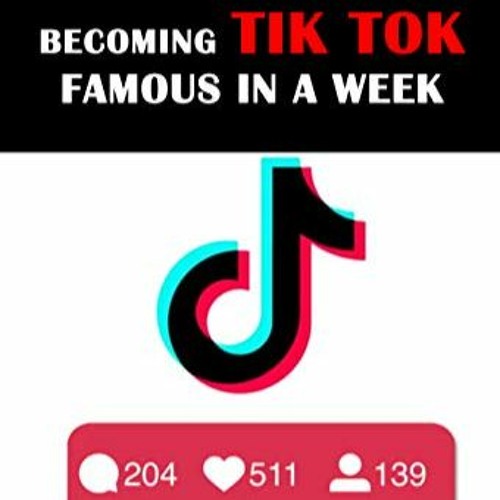In this social media post, the top section features a prominent black banner with the bold, all-caps white text reading "BECOMING FAMOUS IN A WEEK." The phrase "TIKTOK" is emphasized in larger, bold capital letters in red. Beneath this banner, a white background showcases the distinctive TikTok logo, designed as an italicized 'T' with a unique wing-like flourish extending from the cross of the 'T'. This logo appears in a layered combination of turquoise, red, and black colors.

Following the TikTok logo, a bright red banner accents the lower portion of the image. This banner contains three symbols, each paired with corresponding numbers: a conversation bubble with the number "204," a heart icon indicating "511," and a person icon displaying "139." The red banner features rounded edges at the sides, while the bottom corners are sharply defined, creating a dynamic contrast with the rest of the design.